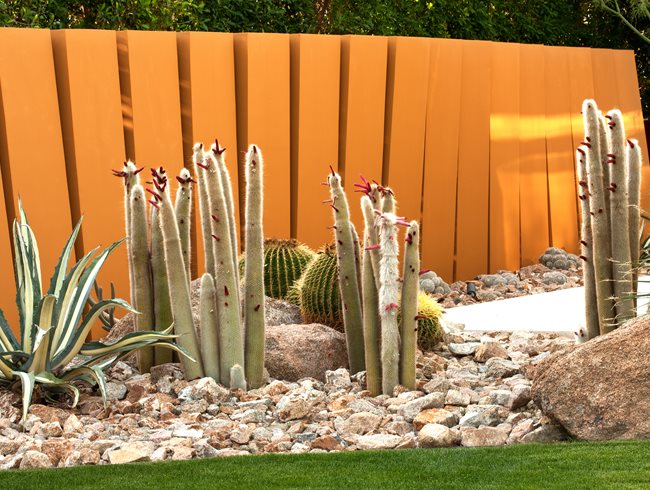The photograph captures an outdoor cactus garden framed by an orange, slatted fence. In the foreground, a thin strip of grass transitions into a bed of white rocks and gravel, which forms the foundation of the garden. The garden boasts a diverse collection of succulents and cactuses, including tall, cylindrical varieties with red buds, and more spherical cactuses adorned with spikes. Among them are plants with spiky green and white variegated leaves. The backdrop of the orange fence, complemented by the greenery of trees peeking over the top, creates a vivid contrast with the rocky terrain and diverse plant life below. This meticulously arranged garden presents a striking scene of desert flora.